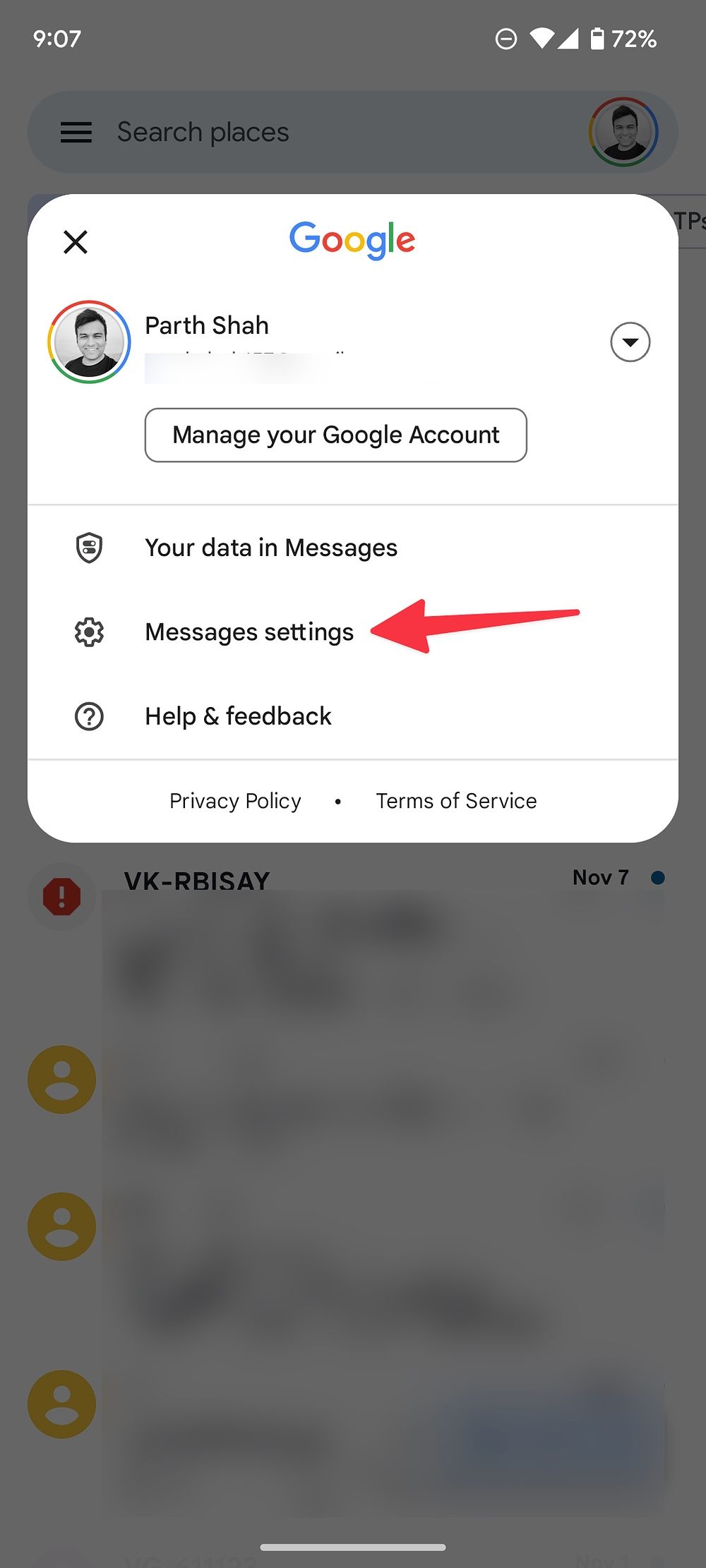The image captures an Android device screen at 9:07 (AM or PM unspecified), with 72% battery remaining, full Wi-Fi signal, and full cellular bars. The phone, presumably belonging to Parth Shah, displays the Google Settings interface, specifically focusing on managing message settings. A red arrow highlights this section, suggesting the image is part of an online tutorial or instructional guide. The background shows a pop-up overlay for message settings atop the main messaging app, possibly Google Mail, indicating Parth is adjusting notification preferences for his messages. The tutorial aims to guide users through customizing these settings for optimal alerts.